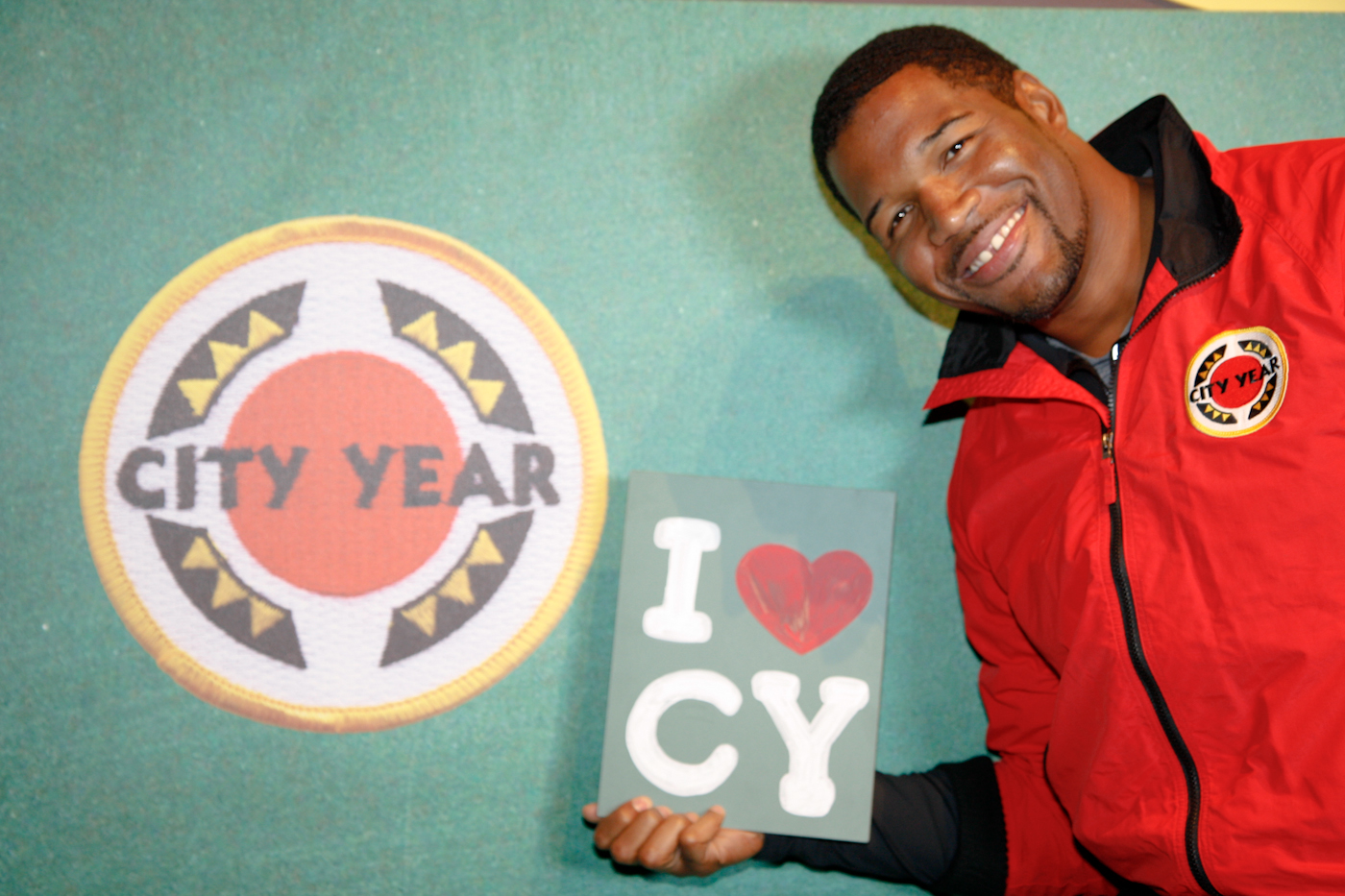The image showcases a vibrant indoor setting centered around a promotional theme for City Year. In the background, there is a primarily greenish-blue backdrop adorned with a large circular logo positioned on the left side. This logo features multiple borders—starting with an outer yellow rim, followed by a white border, a black rim segmented by three yellow triangles, another white section resembling sunrays, and a red central circle. The text "City Year" is prominently displayed within the red circle, making it a focal point in the design.

On the right side of this image stands a man wearing a distinctive red jacket with a black collar, which prominently features the same City Year logo as a patch. The man faces the camera, with his head slightly tilted to the right and his right arm extended at a right angle holding up a sign. This sign, emblazoned with the text "I ♥ CY," is positioned closest to the center of the photograph, drawing immediate attention. The colors within the image balance between shades of green, yellow, white, black, red, and brown, adding to the energetic and cheerful atmosphere, consistent with an advertisement or promotional campaign.